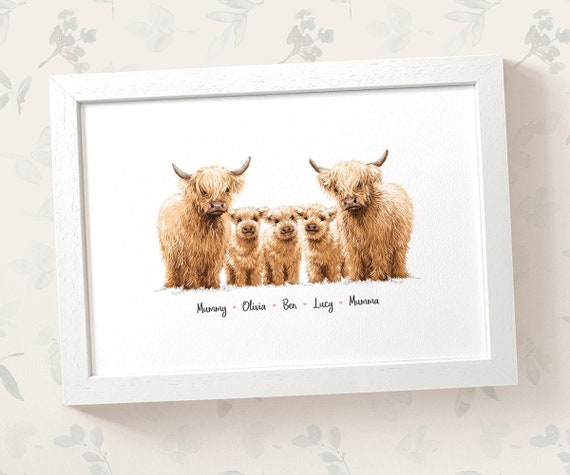A color photograph in landscape orientation showcases a framed art piece against a white wall with a subtle flower motif. The photograph, presented in a white wood frame slightly angled to the bottom left, illustrates a family of Highland cows. This family of furry, horned creatures is composed of two adult cows, one on the left labeled "Mommy" and another on the right labeled "Mama," along with their three calves named Olivia, Ben, and Lucy positioned in the center. All look directly at the viewer, floating against a stark white background. The style is one of photographic representationalism, capturing the realism of the furry family in a whimsical manner. The names of the cows are inscribed in black cursive text below each family member.